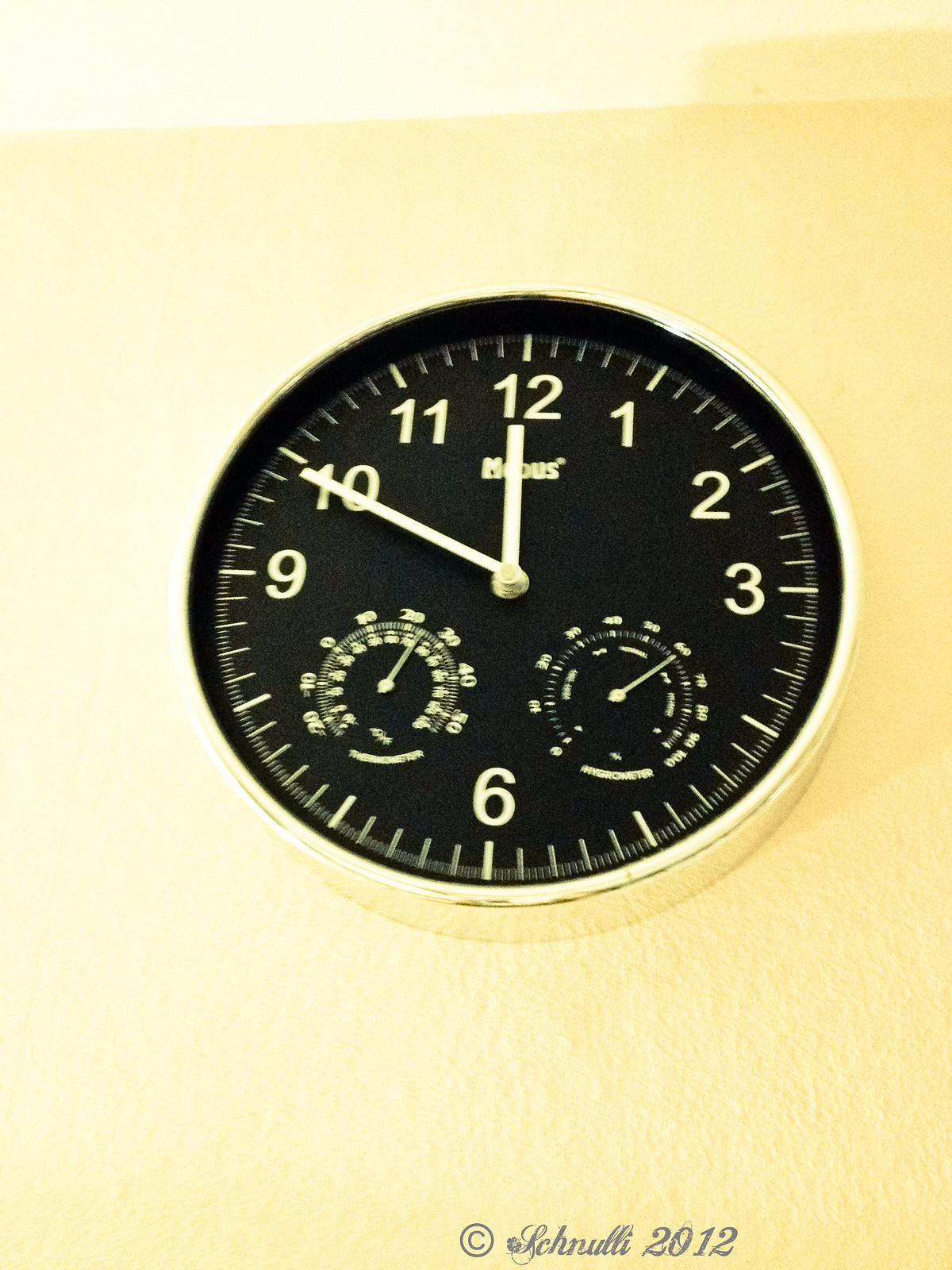A wall-mounted clock displaying the time as 12:50, features of which are complemented by two smaller gauges. One gauge is likely a thermometer, reading approximately 74°F (around 23°C), while the other is a hygrometer, indicating a humidity level of 60%. The clock has a striking design with a black face, white numerals, and a sleek chrome frame. Though the picture is slightly blurry, the overall aesthetic is modern and elegant.